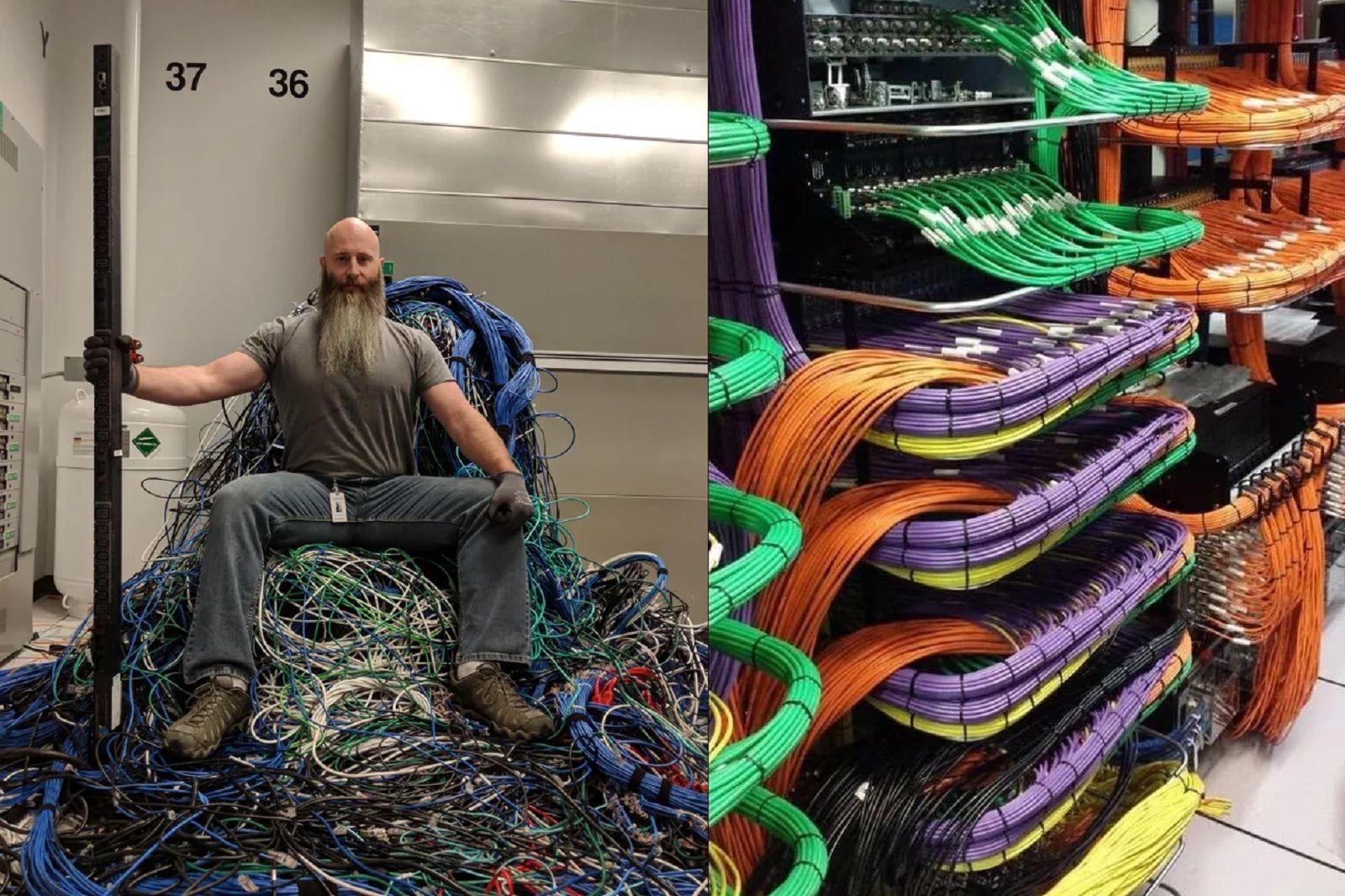The image consists of two distinct, side-by-side photographs in a landscape orientation, each captured in portrait style. The left photograph features a young Caucasian man, likely in his twenties or thirties, with a striking appearance: a bald head and a very long gray beard that extends to the middle of his chest. He is seated on what resembles a throne constructed from a cluster of multicolored wires, reminiscent of a parody of the Iron Throne from Game of Thrones. He is wearing an olive green short-sleeved t-shirt, gray jeans, black gloves, and brown lace-up work shoes. Seated in an industrial indoor setting, he faces the camera and clasps a high black pole with his right hand, extending from the shoulder. Behind him, the setting includes a wall partially covered in white drywall and partially in an aluminum metal partition, with the numbers 37 and 36 visible in black text. A steel chute is seen on the right side within the background, enhancing the industrial ambiance.

The right photograph complements the left by depicting a meticulously organized array of wires in several vibrant colors, including lime green, orange, purple, and yellow. The wires are neatly coiled and stored in bins across six shelves, with purple wires filling the bins and orange wires protruding and hanging over the sides. Above these shelves, a horizontal row of green wires is visible with multiple rows of orange wires behind them. The setting includes a white tile floor, consistent with an indoor environment, likely a network or data server room, as suggested by the organized racks of electronic equipment. Together, these photographs illustrate a cohesive narrative of a man, possibly an IT or networking professional, surrounded by and managing a complex array of wiring systems.